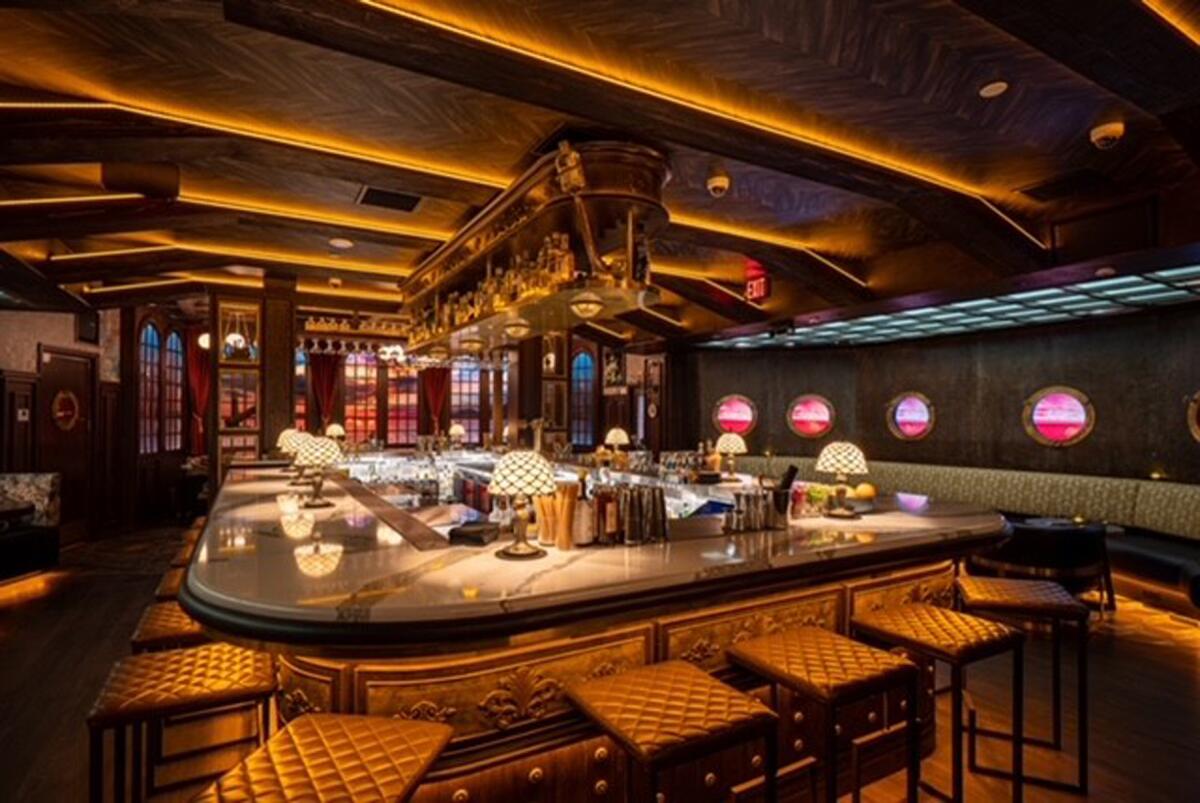The image depicts an inviting yet dimly lit bar and lounge area, possibly within a hotel, featuring predominantly yellow and brown tones. Central to the scene is a large, shiny marble bar, shaped in a square or rectangular configuration, adorned with intricate gold etching along its edges. The bar top, illuminated by elegant Tiffany-style lamps, is both functional and stylish, showcasing several empty glasses and indicating the drink preparation area. Surrounding the bar are numerous tufted, backless stools upholstered in brown leather, their reflective surfaces giving off a yellowish hue due to the strong ambient lighting. Above, the ceiling is crisscrossed with dark wooden rafters, interspersed with discreet yellow lights that add a warm glow to the space. The walls are dark, accented by circle designs in shades of gray and pink, lending an eclectic touch to the decor. On the right side of the image, circular windows and a prominently placed exit sign contribute to a submarine-like vibe. In the background, more traditional windows frame the scene, further enhancing the sophisticated yet cozy atmosphere of this seemingly empty, ready-to-host venue.